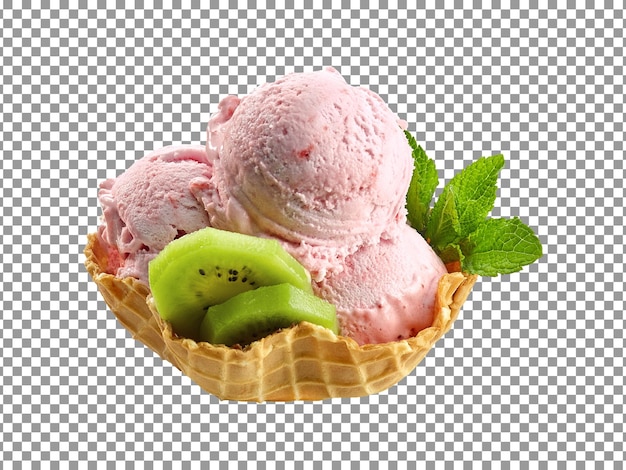The image features a delightful ice cream dessert presented in a bowl made of an edible waffle cone with a light brown, grid-patterned surface. Inside the bowl, there are three scoops of pink ice cream, which could potentially be strawberry or cherry flavored. The scoops are arranged with one on top, one on the left, and one on the bottom right. Garnishing the dessert, to the very right of the scoops, are three leafy green vegetables, adding a fresh contrast. In front of the ice cream, there are two light green kiwi slices, each dotted with black seeds and slightly hexagonal in shape. The entire scene is set against a background featuring a gray and white checkerboard pattern, adding a modern, stylish touch to the presentation.